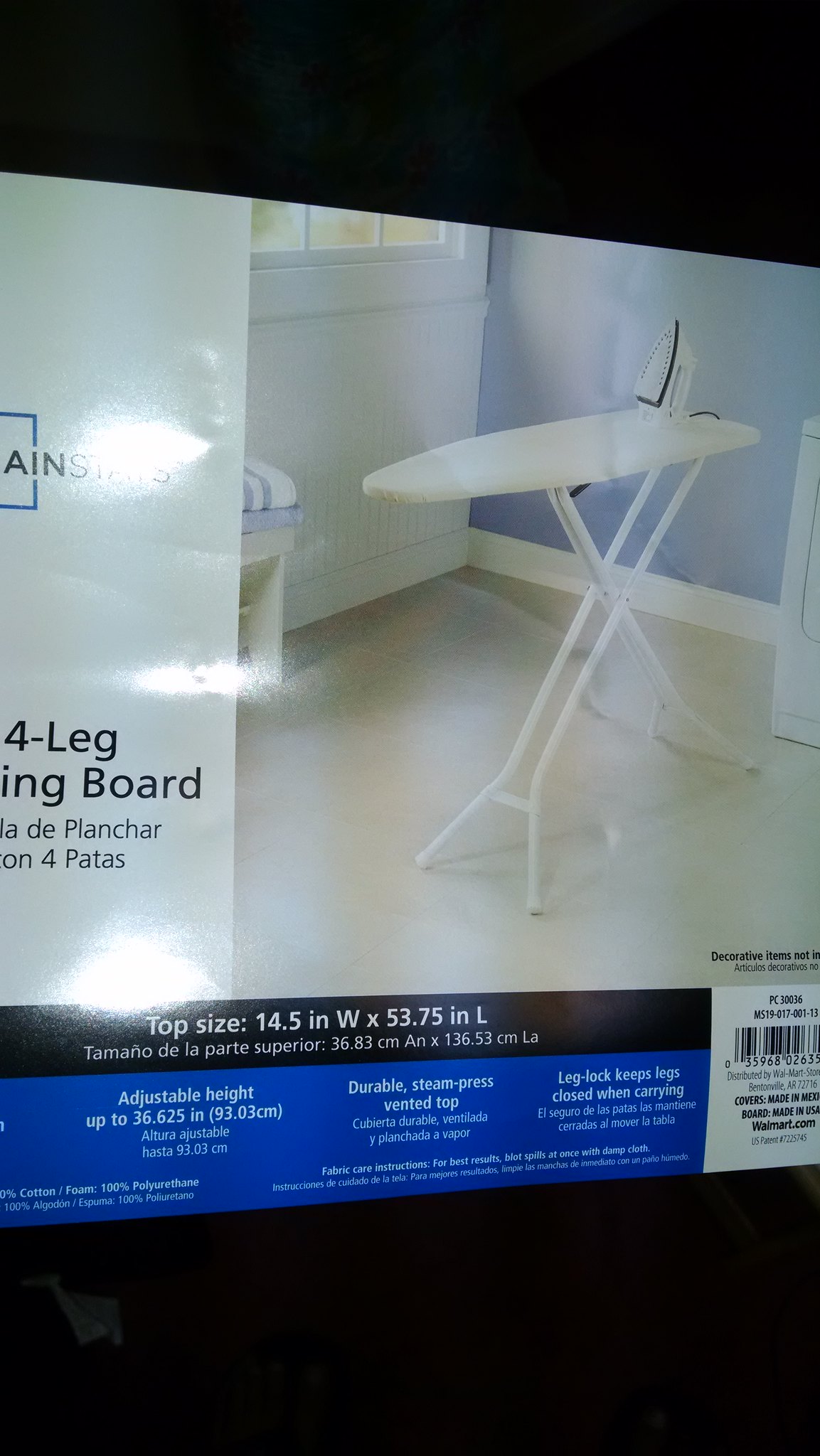The image is a vertical, color photograph of a product label, primarily black, featuring an ironing board advertisement. The photo's perspective emphasizes a portrait layout with significant black space above and below the central object - a carton partially visible within the frame. The carton prominently displays a white ironing board with four fold-out legs arranged in an X pattern, and a white and black iron resting on its backend, facing the 7 o'clock direction. The background scene in the photograph shows a simplistic room setup, including a tan carpeted floor and a blue and white wall, with hints of a window, a piece of a dryer, and a chair.

The label's brand is "Mainstays," although partially obscured, starting with "AIN." Text in a blue rectangle mentions an "adjustable height up to 36.625 inches (93.03 cm)," along with and bilingual details on "durable steam press vented top" and "leg lock keeps closed when carrying." The bottom left features a white ironing board with its dimensions specified in a black strip: "Top size 14.5 inches W x 53.75 inches L" (36.83 cm x 136.53 cm). Additionally, there's a barcode with product care instructions such as "100 percent polyurethane fabric... decorative items not included... covers made in Mexico... board made in USA" and the store name "walmart.com." The overall composition and detailed specifications highlight the key features and usability of the ironing board, standing out against the stark black background.